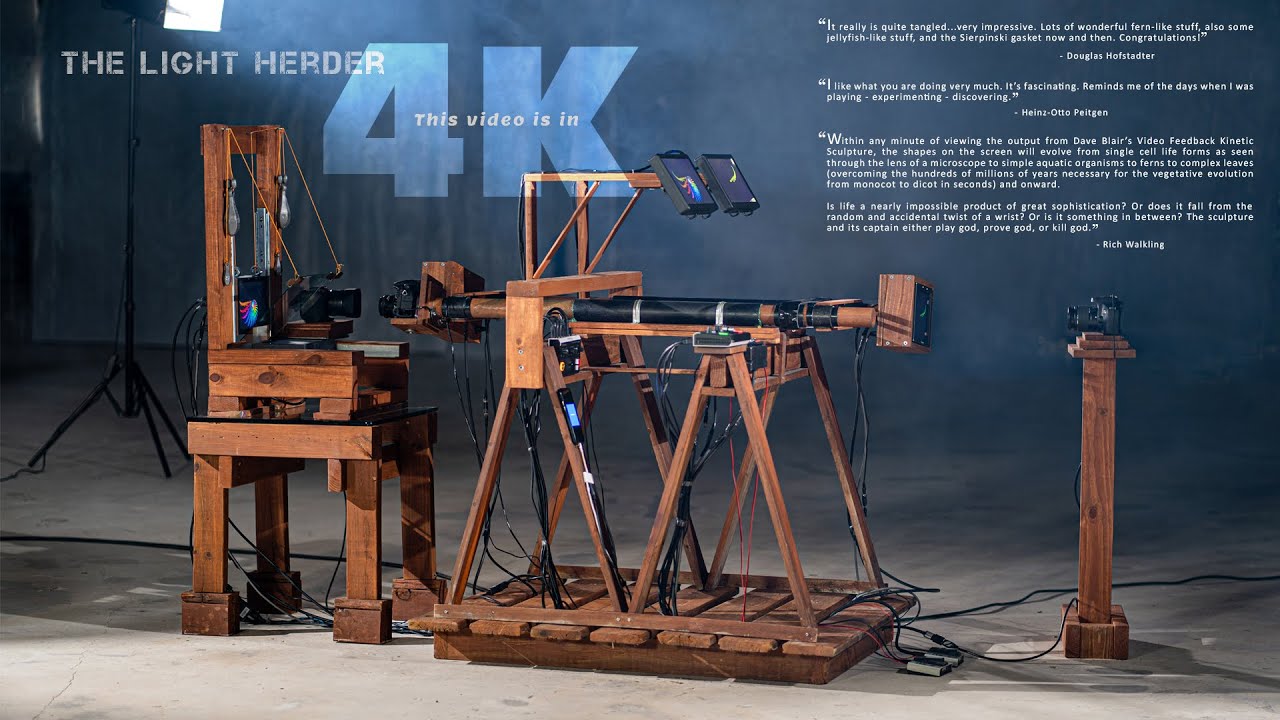This intricate photograph showcases a complex assembly of machinery and electronic equipment, set against a backdrop of a large, industrial space. Dominating the upper left of the image, white text reads "The Light Herder," accompanied by smaller text that states "This video is in," while a prominent "4K" in light blue text sits behind it. In the upper right corner, there are three quotes, though their details and attributions are too small to decipher.

Central to the image is a sophisticated apparatus featuring numerous wooden elements. Wooden racks, shelves, and a stand sustain various mechanical parts, including tubes, wires, and multiple displays. A handheld camera on a wooden pillar is positioned to point towards a square target through a series of interconnected components. The machinery extends in a linear arrangement, leading from the camera to a wooden chair adorned with more equipment. On the left, a light stand illuminates the setup, casting reflections off the equipment, while a blue fabric backdrop contrasts with the gray, concrete-like floor.

The photograph speaks to a blend of traditional craftsmanship and modern technology, utilizing wooden frameworks to support and organize advanced video production tools. The scene is likely part of a staged environment, designed to demonstrate the synergy between analog and digital elements in creating high-resolution 4K video content.